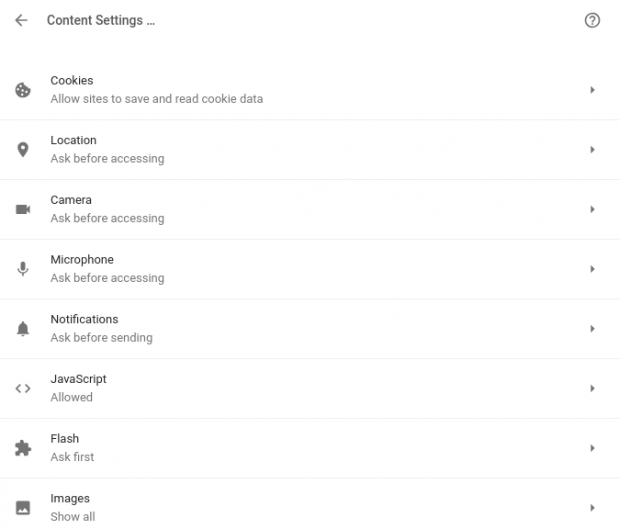The image depicts a web browser's content settings menu against a white background. At the top, black text reads "Content Settings..." with a left-pointing arrow beside it. On the right side, there's a circle containing a question mark. The menu is organized with icons on the left, followed by the name and description of each setting. Each row ends with a right-pointing arrow that can be clicked to open a submenu. Light gray horizontal lines separate the items. The listed settings include:

1. **Cookies:** Allow sites to save and read cookie data
2. **Location:** Ask before accessing
3. **Camera:** Ask before accessing
4. **Microphone:** Ask before accessing
5. **Notification:** Ask before sending
6. **JavaScript:** Allowed
7. **Flash:** Ask first
8. **Images:** Show all

The rest of the menu space is empty.